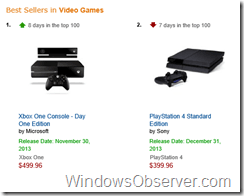This low-quality screenshot appears to showcase a "Bestsellers in Video Games" listing, presumably from an online retailer like Amazon. In the top left corner, a label indicates the category, highlighting the top-ranked items in the video game sector. 

At the number one spot for five consecutive days in the Top 100 is the Xbox One Console Day One Edition by Microsoft. The release date for this console is marked as November 30th, 2013, and it is priced at $499.96. A green arrow next to the listing suggests a rise in ranking.

In the second position, a red arrow signals a decline in ranking for the PlayStation 4 Standard Edition by Sony, which has been in the Top 100 for seven days. This console, released on December 31st, 2013, is available for $399.96.

Both products are represented by corresponding images of the Xbox One and PlayStation 4 consoles. A prominent watermark, "windowsobserver.com," spans the bottom of the screenshot, indicating the source. This scene depicts a ranking system similar to what users might encounter while browsing highly rated products on platforms like Amazon or eBay.